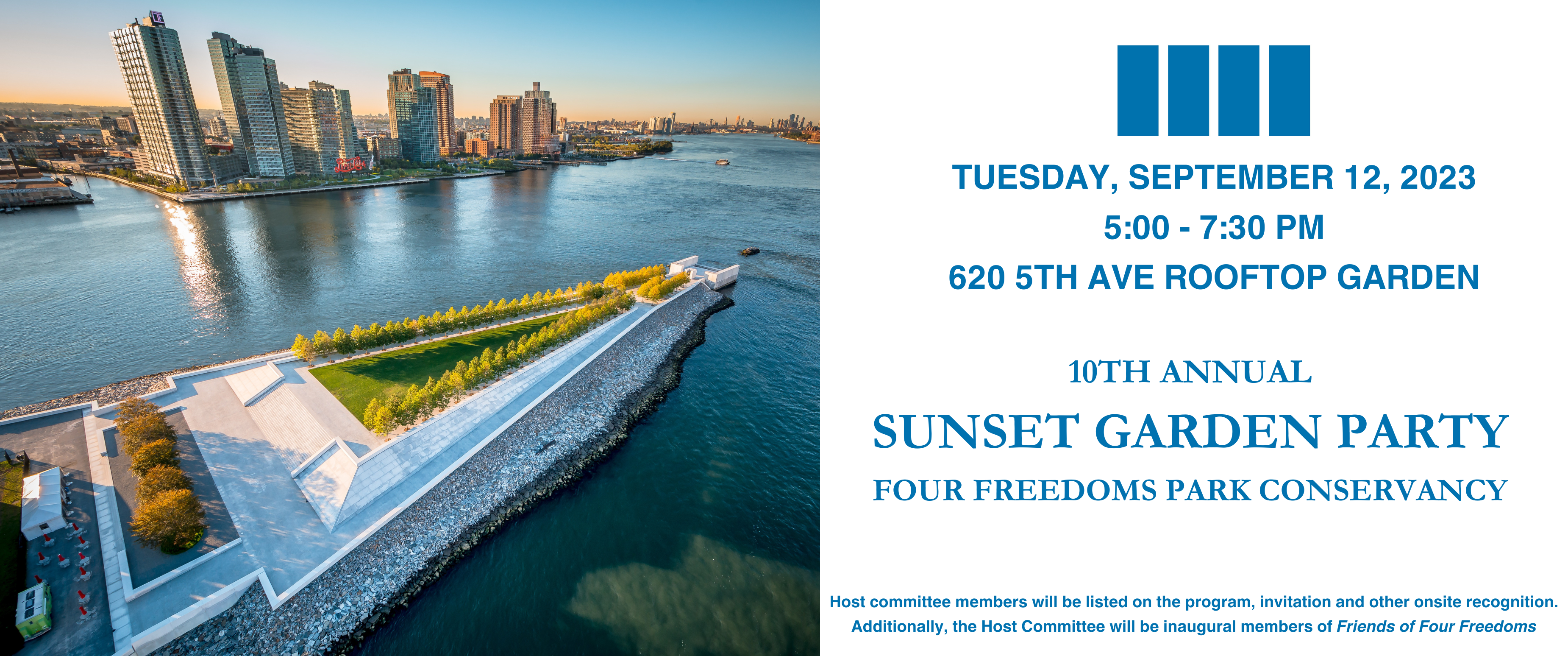This aerial photograph captures a scenic view, likely near Manhattan, from an island area looking towards the city. On the left side of the image, a man-made triangular jetty extends into a waterway, featuring landscaped areas and a low-level cement structure. Surrounding the jetty is a lush park or memorial adorned with trees, and a parking lot is visible at the edge of the frame. In the background, the cityscape dominates, with five prominent high-rise buildings and smaller structures under a clear blue sky. On the right side of the image, text in cornflower blue on a white background announces an event: "Tuesday, September 12, 2023, 5 p.m. to 7.30 p.m., 625th Avenue Rooftop Garden, 10th Annual Sunset Garden Party, Your Freedom Park Conservancy." It specifies that host committee members will be recognized in the program, invitation, and on-site, and will become inaugural members of the Friends for Freedom. The contrasting elements of nature and urban architecture, coupled with the event details, make this image both inviting and informative.